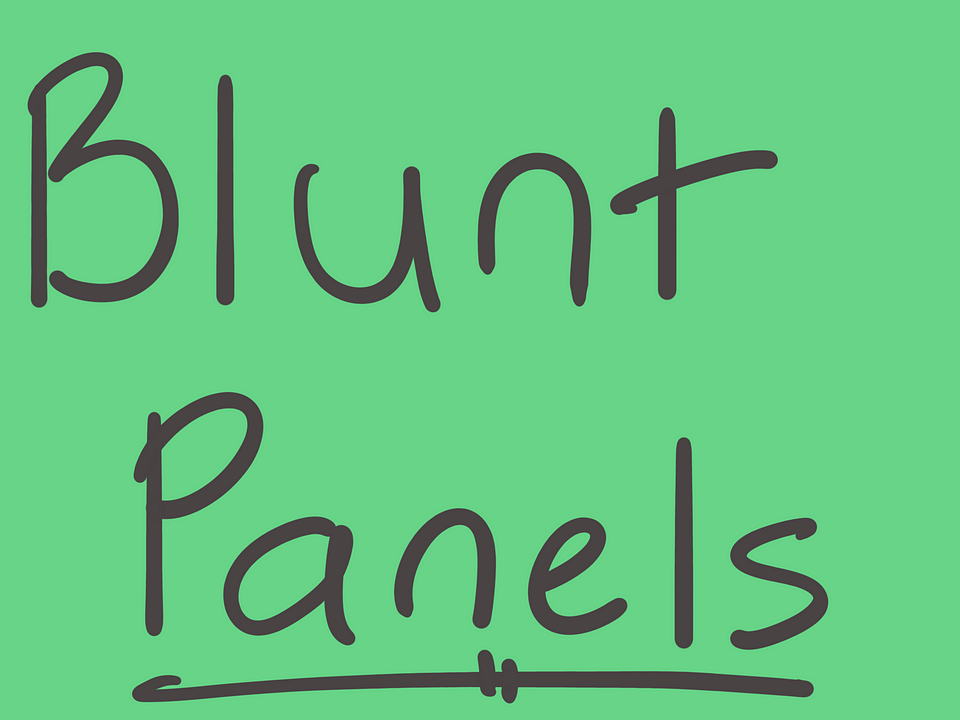The image depicts a simple, pastel green square, measuring approximately 6 by 6 inches, with the phrase "Blunt Panels" written in large, dark, handwritten-like text that resembles the Comic Sans font. The top word "Blunt" has a capital 'B' followed by lowercase letters, while the bottom word "Panels" has a capital 'P' followed by lowercase letters. The word "Panels" is underlined by a single horizontal line with two vertical lines intersecting it in the center. There are no other identifying marks, images, or information present in the image, creating a minimalist and uncluttered design.